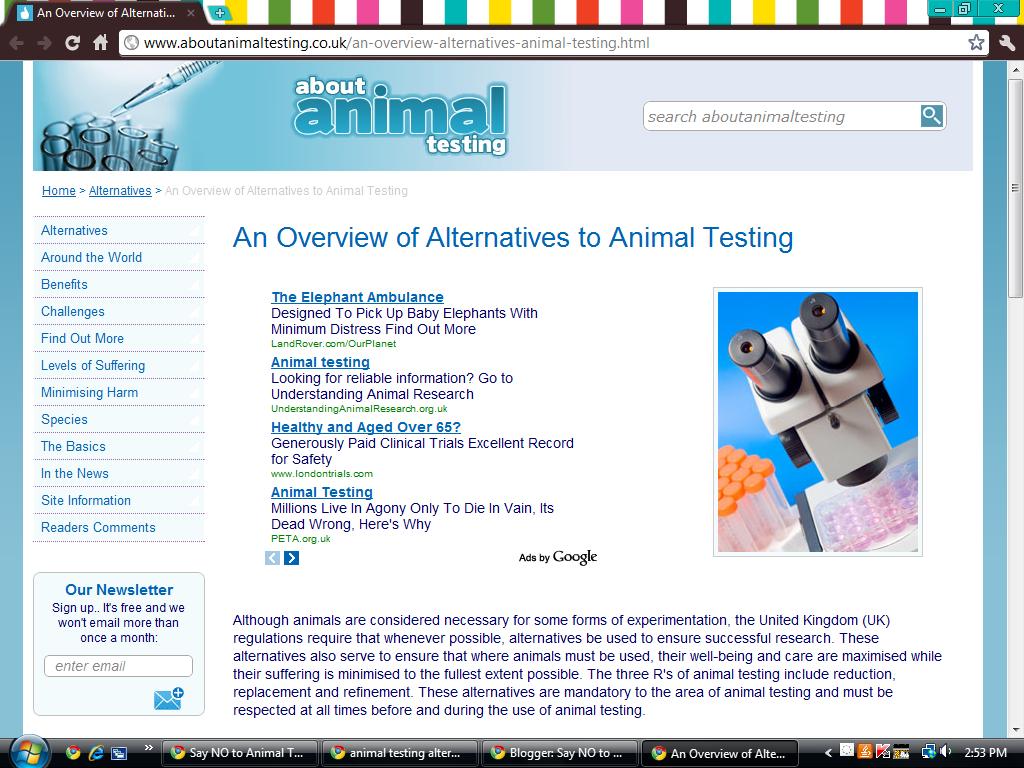The image captures a detailed snapshot of a website named aboutanimaltesting.com, displayed in the Google Chrome browser. On the right side of the webpage, there is a prominent picture of a white microscope. To the left, the website features a navigation menu with various categories in blue font, including "Alternatives Around the World," "Benefits," "Challenges," "Find Out More," "Levels of Suffering," "Minimizing Harm," "Species," "The Basics," "In the News," "Site Information," and "Readers Comments." At the very top of the webpage, a search bar is visible. The browser window shows additional contextual elements, such as the Windows logo located at the bottom left of the screen, which is a wavy square divided into four colors: green, blue, yellow, and red. The taskbar at the bottom reveals that four instances of Google Chrome are open.